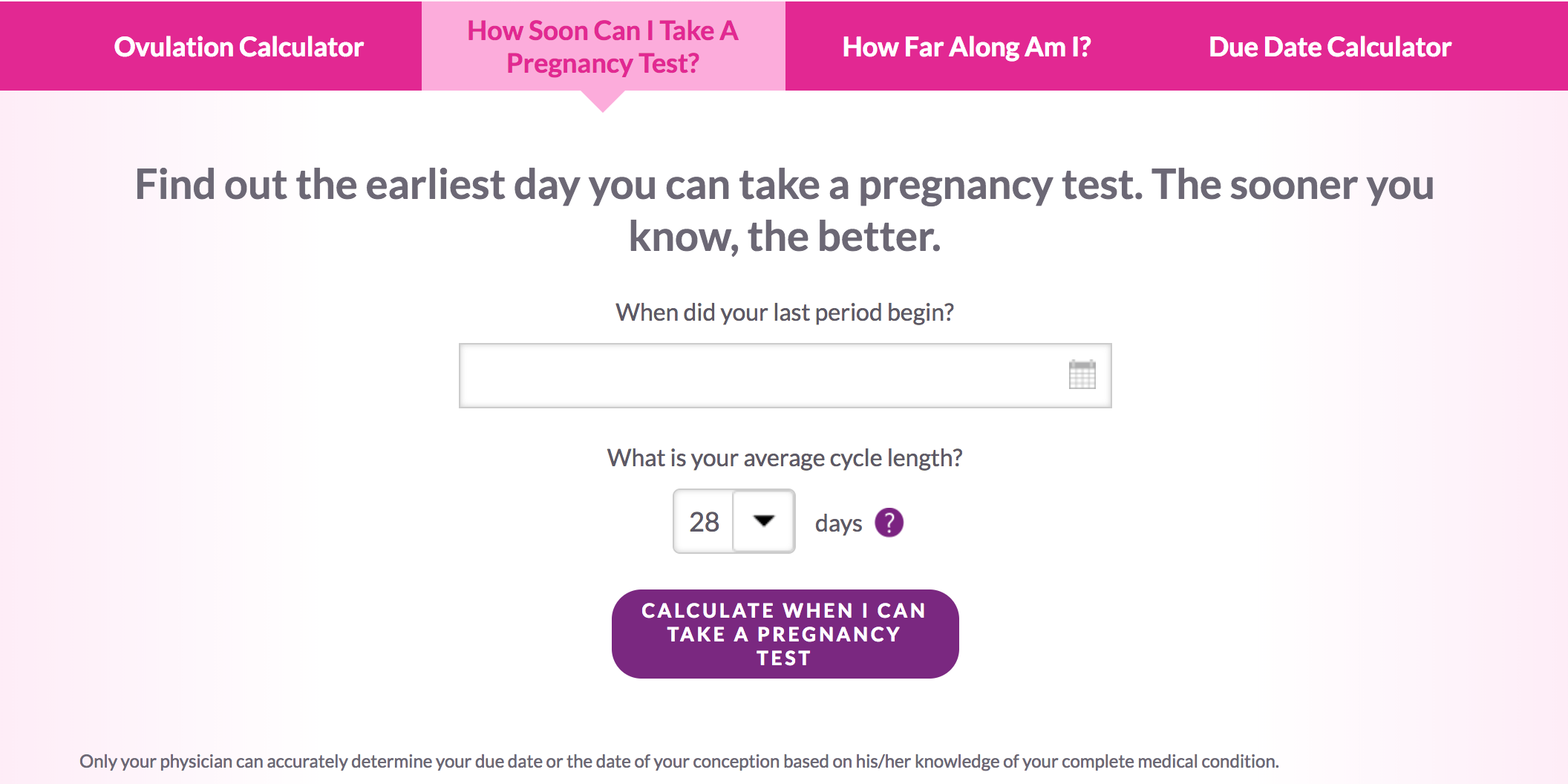The website for pregnancy tests features a prominent dark pink border at the top, where various tools are listed, including an ovulation calculator, a guide on how soon one can take a pregnancy test, information on how far along a pregnancy might be, and a due date calendar. 

Below the header, the main body of the website offers guidance on determining the earliest possible day to take a pregnancy test, emphasizing that early knowledge is advantageous. A central search bar prompts users to input the start date of their last period and their average cycle length, featuring drop-down menus and a calendar for easy selection of dates.

A highlighted purple button with rounded corners, conspicuously placed in the middle of the page for easy visibility, invites users to calculate when they can take a pregnancy test. Despite the tools provided, the website clearly states that only a physician can accurately determine a due date or the date of conception, based on comprehensive medical knowledge of the individual’s condition.